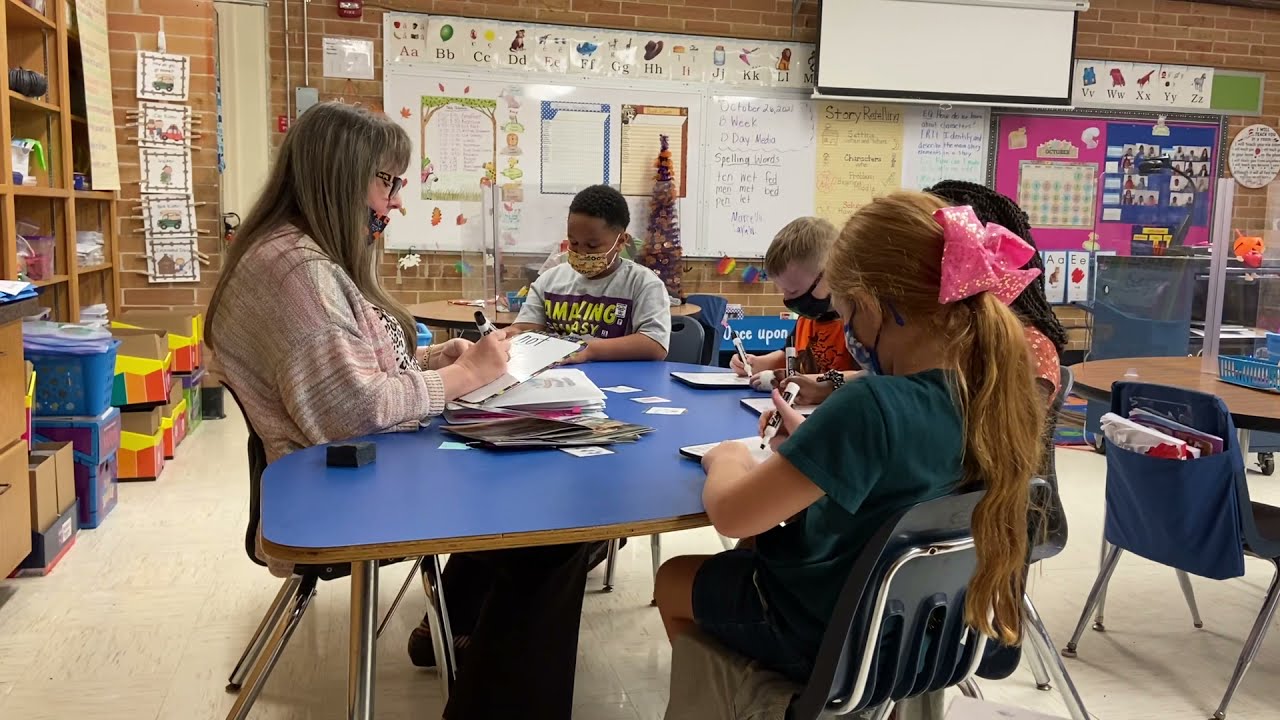The image depicts a classroom scene, most likely in a middle or elementary school setting, perhaps for fifth or sixth graders. The room features a distinctive blue table, low to the ground, around which sit a female teacher and four students—two girls and two boys. One of the girls is identifiable by a pink ribbon in her hair. They are all engaged in an activity, writing on handheld whiteboards with Expo markers, and every individual is wearing a mask, suggesting the image was taken during the COVID-19 pandemic. The classroom environment includes brick walls and a white-tiled floor. The room is well-equipped with educational materials, including stacks of papers, little cards, colorful posters, the alphabet displayed on the walls, a projection screen, numerous whiteboards, and a clock. Additionally, there are various totes filled with school supplies and learning materials positioned around the room. This snapshot captures a focused learning session in a vibrant and well-organized educational space.